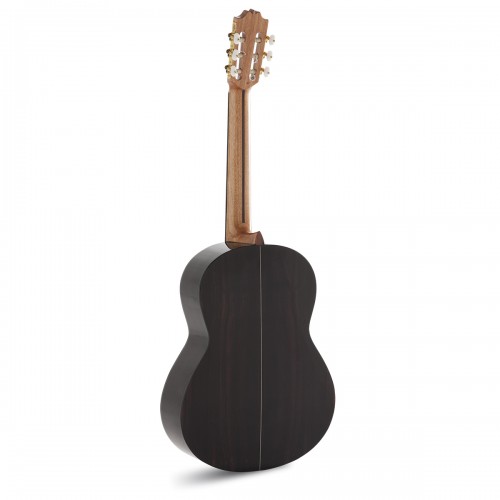The image showcases a standard acoustic guitar photographed from the back against a white background, drawing particular focus to the instrument itself. The body of the guitar is a very dark brown, almost black, and features a noticeable crack down its back. Its neck is made of a lighter, natural wood that contrasts with the darker body. The guitar is slightly angled away from the camera, so the front is not visible. The tuning pegs are a combination of silver and white, with the tuning pieces described as white and gold. The lighting is designed to highlight the right-hand side of the guitar, casting a shadow underneath and slightly to the left, suggesting the light source is positioned overhead and to the right. The composition and negative space indicate that this is likely a product image, similar to what one might find on a retail site like Amazon, intended to show the guitar from a different angle as part of a series of supplemental images.